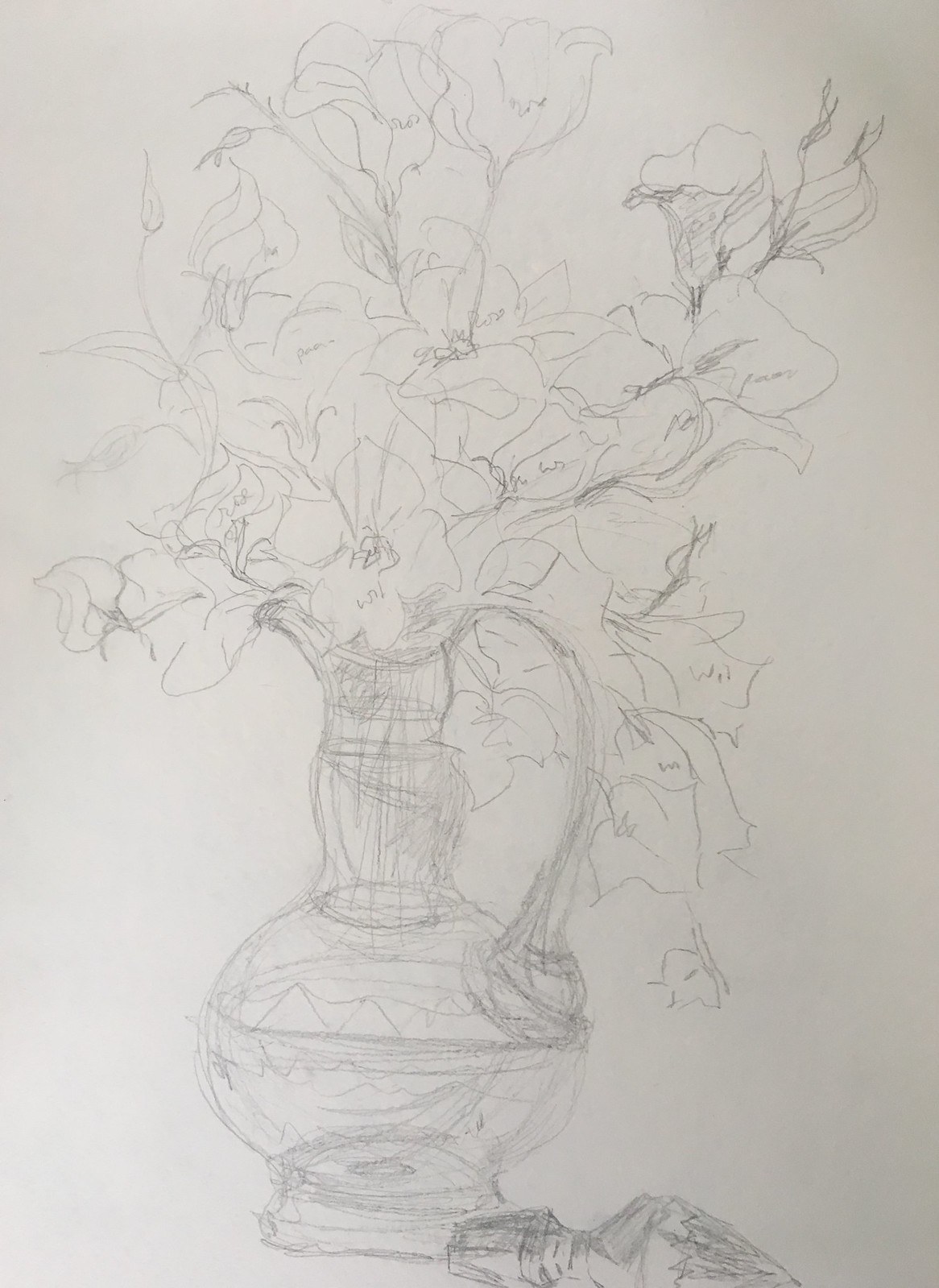This pencil sketch captures a detailed image of a tall, urn-like vase positioned in the bottom center of a white background. The vase features a round body with a rectangular base, a narrow neck forming a spout on the left, and a long handle that extends from the top left down to the horizontal center line of the vase. Partially shaded, the vase is filled with a large bouquet of lightly outlined flowers and greenery, which appear to have four petals each. The flowers are arranged in a sketchy, almost unfinished manner, extending upwards and outward from the vase, giving the sense of a dense, overflowing bouquet. There's an additional horizontal object, possibly a glass stopper, positioned to the right of the vase. The overall composition is vertical, filling most of the white background with its artistic and somewhat incomplete depiction of the floral arrangement.